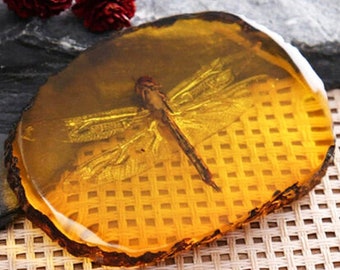The image depicts a low-resolution, slightly blurry photo of a piece of amber, which houses a large, ancient dragonfly. The amber, golden yellow in the center and deeper brown around its rough, jagged edges, is oval-shaped and smooth in the middle, with a combination of flat and spherical contours. The dragonfly is positioned inside the amber with its head oriented towards the top left and its tail extending to the bottom right. Its four clear wings are fully extended alongside its long, narrow brown body, laying flat as if it has been preserved for centuries. The amber piece is placed on a light-colored, wicker or caning material, adding a textured backdrop. The outdoor setting of the image suggests the specimen might have just been collected by a researcher for examination. In addition to the wicker surface, two red fuzzy objects are visible in the top left corner, and a stone surface can be seen in the top right, adding context to the environment in which the photograph was taken.